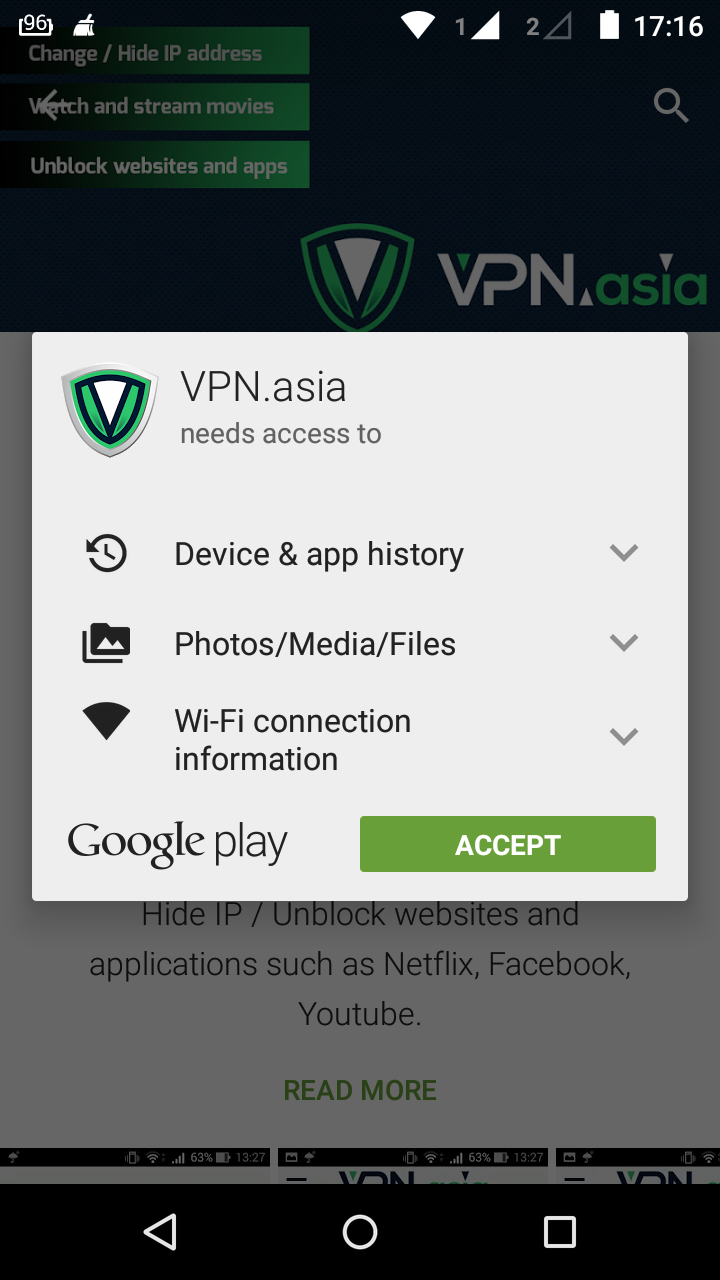This mobile screenshot captures the interface of a website called VPN Asia, showcasing a pop-up centered on the screen. The pop-up is a prominent white square box. At its top, the text "VPN Asia needs access to" is displayed, accompanied by the VPN Asia logo positioned in the top left corner. 

In the main section of the pop-up, there's a series of three icons aligned to the left, each corresponding to a dropdown menu on the right. The icons represent options titled "Device and app history," "Photos, media, and files," and "Wi-Fi connection and information." Each dropdown allows the user to select whether to permit or deny access.

At the bottom of the pop-up, "Google Play" is written in gray letters on the left. In the bottom right corner, a large, green "Accept" button with white lettering stands out, prompting the user to proceed.

In the background, faintly visible behind the pop-up, is the VPN Asia website. The top of the page features a black border with "VPN Asia" centered within it. Below this header, the website's content appears against a white background.